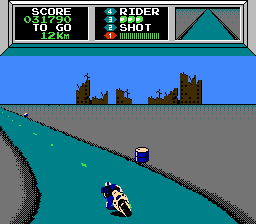This vibrant pixel-art screen grab from a video game captures a dynamic scene of a rider on a bright yellow motorbike cruising down a two-lane green road. The road is flanked by gray shoulders and stretches into the distance, where it meets a stark black city skyline silhouetted against a clear blue, cloudless sky. At the top of the screen, game stats are displayed: the score reads 031790, with 12 kilometers remaining for Rider Three. Additionally, three yellow circles—likely representing indicators or power-ups—adorn the upper section of the frame, with two of them evidently "shot" or activated.